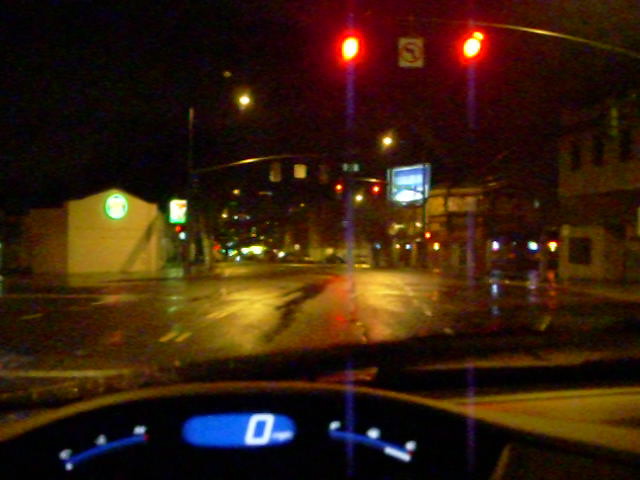An image captures the view from the inside of a stationary car, with a portion of the dashboard visible displaying bright blue and white illuminated lights, including a prominent '0' indicating the car is stopped. The windshield shows streaks from the rain, highlighting the ongoing downpour. Outside, through the rain-streaked window, a red traffic light is visible along with a "No Left Turns" sign. The wet pavement glistens under the streetlights, adding to the scene's rainy atmosphere. Further in the background, additional streetlights illuminate the area, and a building on the left showcases a white sign with green trimming. On the right side of the frame, there are buildings with lit windows and a brightly lit billboard. The overall scene exudes a rainy, nighttime urban environment.